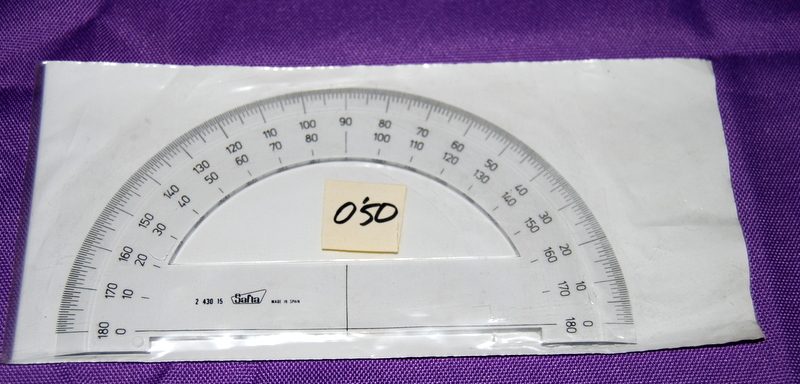The image depicts a purple fabric that borders the edges of the picture. At the center lies a solid white rectangular envelope or packaging material. Placed atop this white surface is a clear plastic protractor, characterized by its semi-circular shape and functions to measure angles. The protractor features degree markings ranging from 0 to 180 degrees in both directions. At its center, where the protractor forms an open arc, there is a yellow post-it note with the handwritten number '0'050, denoted with an apostrophe between the first '0' and the '5'. This note is perfectly positioned within the open central part of the protractor, giving the entire composition a neatly organized appearance.